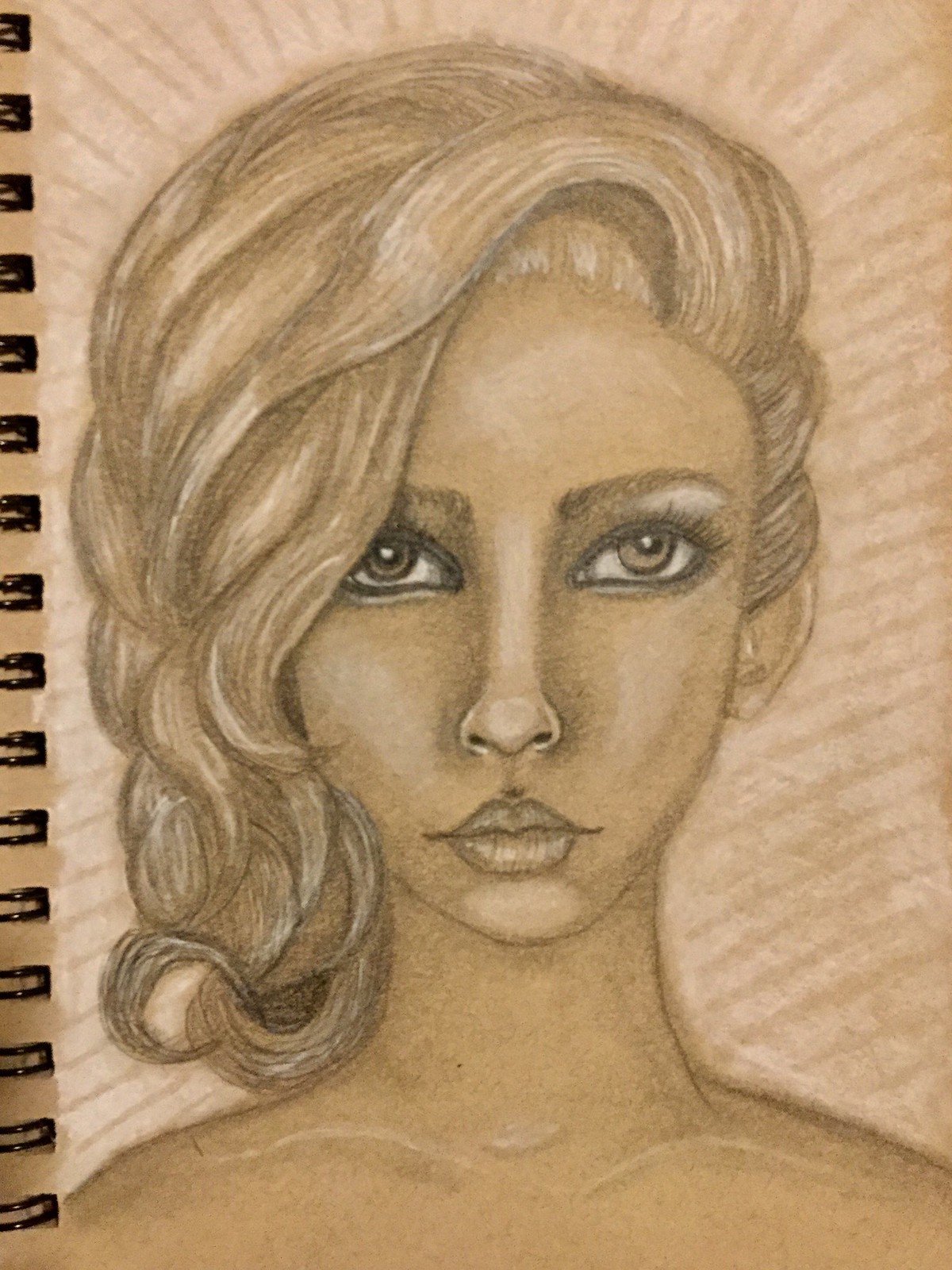This detailed drawing portrays a female figure, set against a pinkish background with radiating lines originating from the head. The subject has neck-length, blonde hair that is parted to their right side, with bushy, darker eyebrows. The eyes appear to be a blend of green and hazel, adding depth to the face which is depicted with a medium skin tone. The nose is narrow, thin, and delicate at the tip. The medium-sized lips are shown with careful detailing that suggests they are chapped or lined. The neck is smooth, leading to a visible top collar area that hints at a tube top style, devoid of any straps. The artist has meticulously rendered the shoulder outlines and the natural neck indentations, adding a realistic touch to the overall composition.